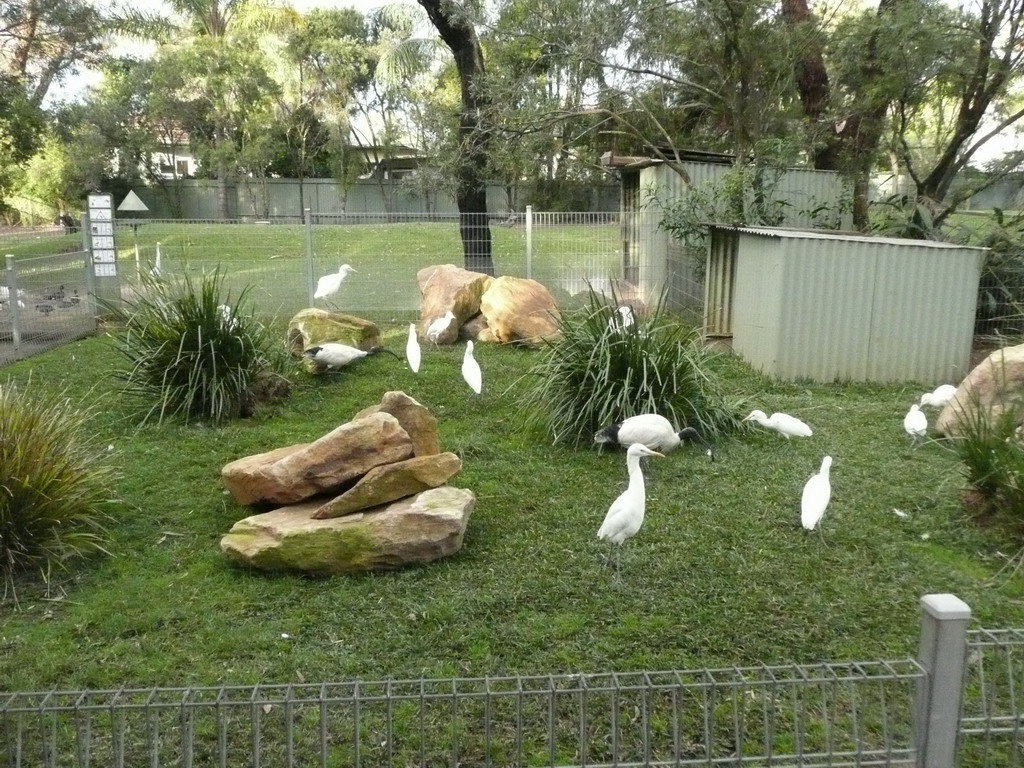The photo captures a meticulously landscaped, fenced-in yard, likely within a zoo or animal sanctuary. The foreground features a small gray metal fence, while a larger white fence with unreadable signage encloses the area in the background. The yard is filled with white birds, possibly ducks, all walking around the lush green grass and pecking at the ground. These birds are surrounded by brown rocks and well-manicured bushes. Dominating one side of the enclosure is a tin duck house with an open door, presumably serving as shelter for the birds. The area includes two sheds with gray siding: a shorter one inside the fence and a taller one outside. Additionally, there are four tall grasses flanking the sides, and multiple trees scattered throughout the yard, adding to the serene setting. The overall scene is vibrant and green, enhancing the peaceful ambiance of the outdoor space.